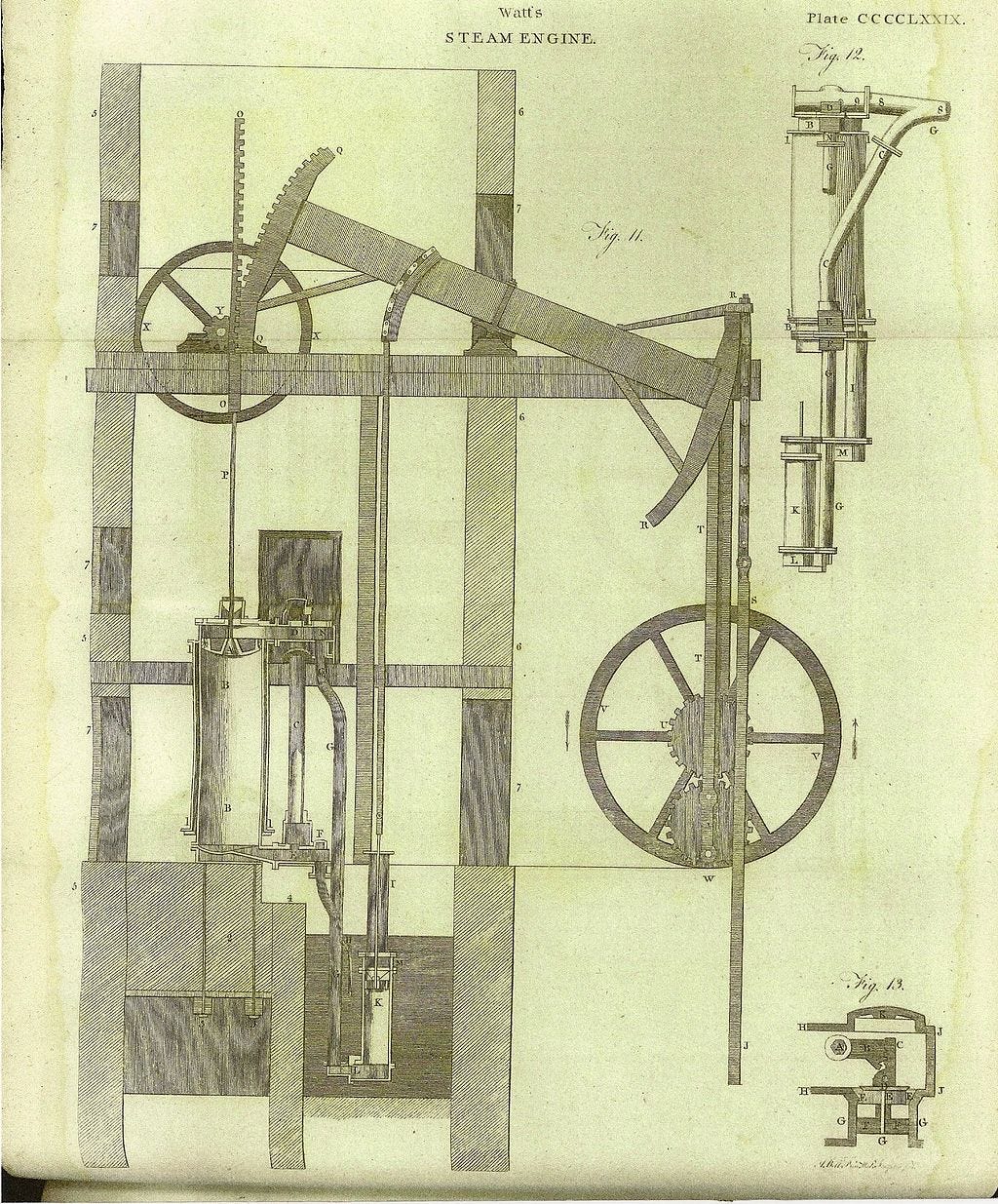This is a black, white, and gray hand-drawn blueprint of Watt's steam engine, labeled as "Plate CCCCLXXIX." The image has a detailed depiction of the steam engine, elucidating various mechanical components such as circular wheels, cranks, levers, and vertical and horizontal projections. The intricate drawing employs uppercase letters to label each piece, resembling a technical blueprint an architect might create. Featured prominently are figures 11, 12, and 13, indicating different aspects and details of the engine. Figure 11 captures the main body of the steam engine with a complex arrangement of geometric shapes and metal contraptions. Figure 12, located on the right, depicts a cylindrical component that resembles an air pump with an attached bar. Figure 13 in the bottom right highlights a network of interconnected bars. The base of the engine appears to be made of wood or metal. The paper of the illustration is yellowed and exhibits signs of water damage around the edges, suggesting it's from an old book. The image is not a realistic photo but a meticulous, architectural-style drawing, replete with labeled parts and a clear depiction of the steam engine's structural intricacies.